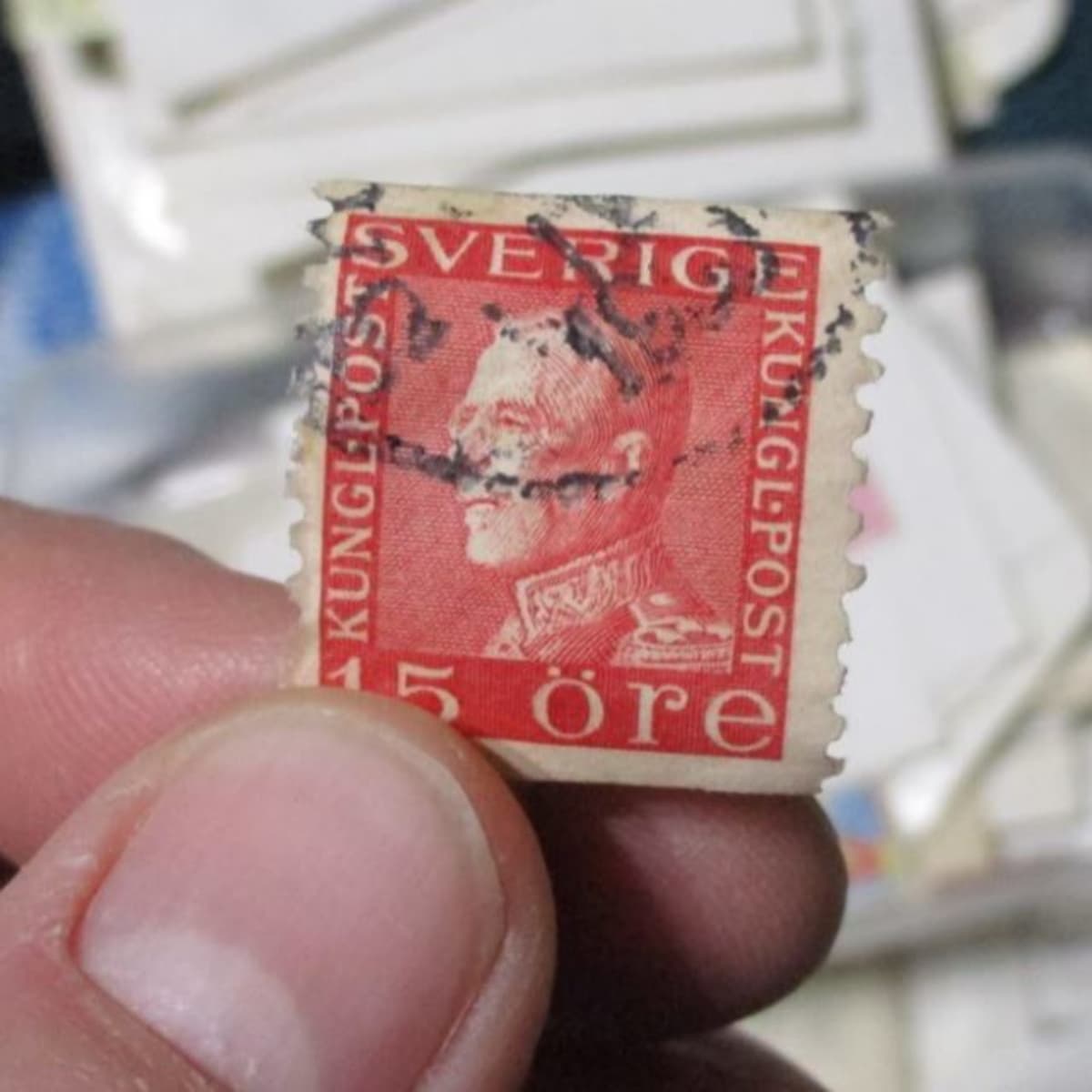In the image, a person is carefully holding an old, red stamp between their left thumb and forefinger, showcasing well-groomed fingernails. The stamp, prominently centered in the picture, features a white border with the word "SVERIGE" in white letters positioned at the top against the red background. On both the left and right sides, the vertical letters spell "K-U-N-G-L POST." At the bottom of the stamp, "15 ÖRE" is inscribed, also in white. The red backdrop of the stamp hosts an intricate portrait of a regal figure, likely a king, characterized by short hair, glasses, and a uniform with a high collar and epaulets on the left shoulder. The stamp bears a black cancellation mark, partially revealing the number "16," further emphasizing its used status. The background of the image is blurred, drawing attention to the detailed elements of the stamp and the holder's meticulously clean fingertips.